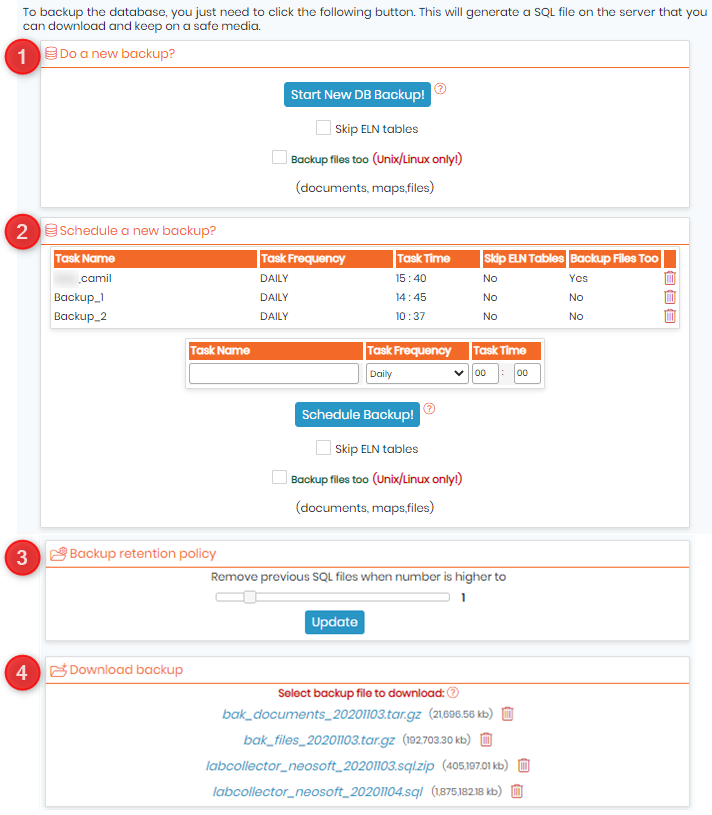**Descriptive Image Caption:**

The image depicts the steps necessary to back up a database. A red arrow highlights a crucial button that initiates the backup process. Clicking this button generates a .sql file on the server, which can be downloaded and saved.

Following this, the user should switch to a straight VLN table layout to manage backups. The instructions then emphasize submitting the generated backup file through the 'unix-linuxonly.com' portal. The process involves navigating to the SQL files section labeled 'sqlfiles2', scheduling the backup and selecting specific options in the interface.

Key fields to be configured include setting the backup frequency to daily and specifying times such as 15:40, 14:45, and 10:37. The user should select options for VLN tables and backup files, noting a particular emphasis on a blue rectangle button for scheduling the backup.

Additionally, details on the backup retention policy are described, such as removing previous SQL files when their count exceeds a certain threshold. The user interface contains a bar labeled 'update', with options to download the latest backup files in various formats like .tar.gz and .sql, dated between 20200103 to 20201103, from a system identified as 'Labcollector Neosa'.